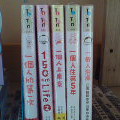A tiny, slightly blurry photo showcases the spines of five books or DVD cases, aligned side by side, prominently featuring Asian characters in bright red on a white background with black text. The top portions of the spines are color-coded—green, pink, yellow, green, and a possibly green or gray hue. Each item appears to be part of the same series, likely a show, although specific titles are in Chinese or Japanese and hard to decipher. Notably, the number "15" in Arabic numerals and the word "life" in English are also visible. The background is darker, contrasting with the brightly colored items, showing a partially open white door, a soft beige wall, and a fancy rug towards the bottom half. The overall setting hints at a room with muted lighting.